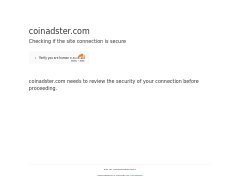The image is a diminutive screen capture from the website coinadster.com. Dominated by a black text on a stark white background, the text at the top reads, "coinadster.com - check if the sheet connection is secure." Directly below this is an orange icon accompanied by an unreadable text. Further down, another line of black text states, "coinadster.com needs to receive the security of your connection before proceeding." Beneath this message lies an expanse of white space. At the very bottom, there is an ultrafine black text that is difficult to decipher, separated from the main content by a faint gray bar. Near the orange icon, there appears to be a small arrow or bullet point, adding a subtle touch of visual punctuation to the text.